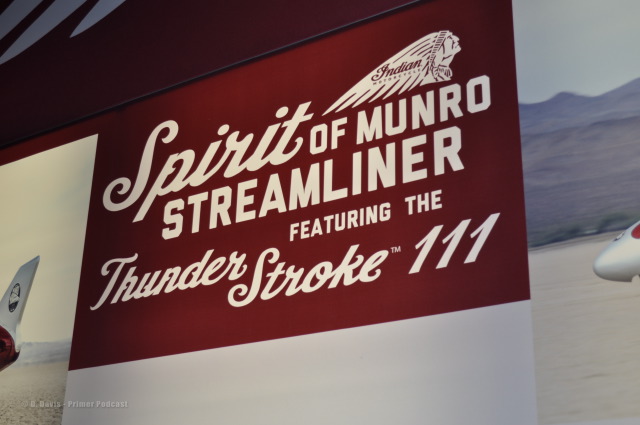This horizontally-oriented photographic image captures an indoor scene featuring a prominent, dark red banner that reads "Spirit of Monroe Streamliner featuring the Thunderstroke 111" in white lettering. The phrase "Spirit" is written in script while "of Monroe Streamliner" and "featuring the" are in block font, and "Thunderstroke 111" is in script with a trademark symbol. To the top right of the banner, there is a graphic of an Indian chief with a long headdress, looking upward, with the word "Indian" written across the feathers. Behind the banner, on the right, the image partially reveals the tip of a silver airplane nose against a mountainous background, and on the left, the white tail of another jet airplane is visible. The banner appears to hang from a dark ceiling with a grayish hue, and underneath it lies a broad white band. The overall setting is dimly lit, enhancing the contrast between the deep red of the banner and the surrounding elements.